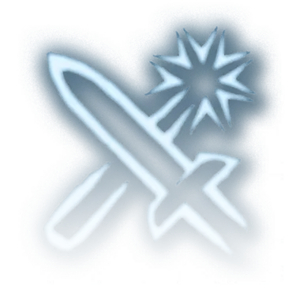The image depicts a stylized depiction of two weapons crossing each other, almost forming an 'X'. Both weapons exhibit a vibrant glow, reminiscent of neon lights, casting an icy blue luminescence around them. The primary weapon at the forefront is a sleek sword, characterized by its sharp blade and pointed tip. Below the sword and crossing it at a diagonal angle is a more ambiguous weapon designed like a spiked mace, with a striking feature of a spiky, star-shaped head filled with numerous needle-like spikes attached to a rectangular handle. The weapons are rendered in shades of gray and white, giving them an x-ray-like appearance, with the icy blue glow accentuating their forms against the contrasting background. This composition of crossed weaponry, outlined in light blue and bordered by white, creates a stark and captivating emblematic image.